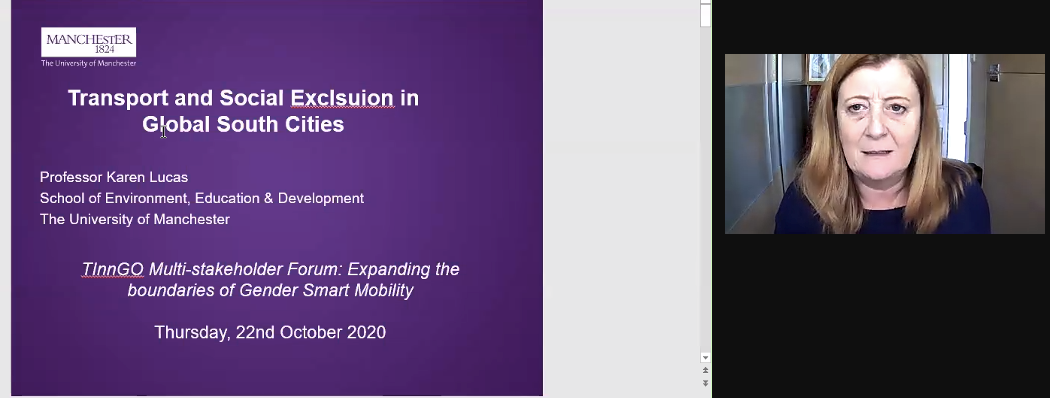The image portrays a wide web application interface resembling a Zoom session. On the left side of the image, there is a purple slideshow with a title in white text reading "Transport and Social Exclusion in Global South Cities," with the word "Exclusion" underlined in red as if by a spellchecker. Below the title, it lists the speaker as "Professor Karen Lucas, School of Environment, Education and Development, the University of Manchester." The slide also includes information about a "TINGO Multistakeholder Forum: Expanding the boundaries of gender-smart mobility," dated "Thursday, 22nd October 2020." At the center of the image, there is a large, empty white block. On the right side, the image features a black rectangle containing a video feed of an older white woman with long blonde hair, wearing a navy blue shirt, appearing to use a webcam. This setup suggests she is participating in the session, likely as Professor Karen Lucas.